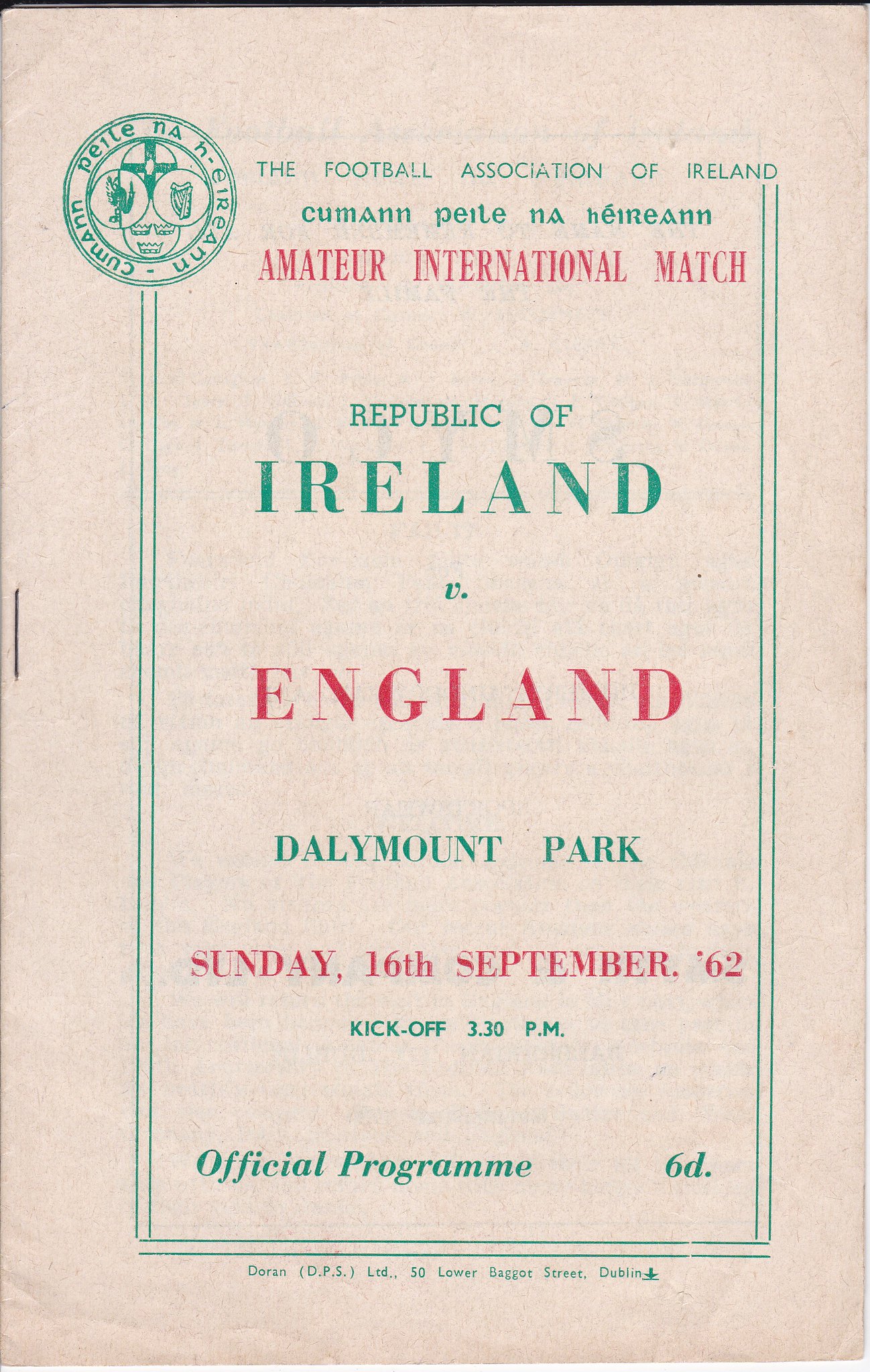The image depicts an old cover page for an official football match program from over 60 years ago, dressed in striking red and green text—the national colors of Ireland. The background is a plain tan or cream color, framed in green, with a visible staple in the middle-left, holding the pages together. The program is titled "Football Association of Ireland, Cumann Píl-ne-Hart," detailing an amateur international match between the Republic of Ireland and England at Daly Mount Park on Sunday, September 16th, 1962, with a kick-off at 3:30 p.m. The words "Ireland" and "England" are in capital letters, with "Ireland" highlighted in green and "England" in red. At the top, a small emblem of the match is visible. The program was printed by Doran DPS Ltd, located at 50 Lower Baggot Street, Dublin, and it was sold for 6D. The design is simple yet evocative of the era, capturing a significant sporting event from Ireland's amateur football history.